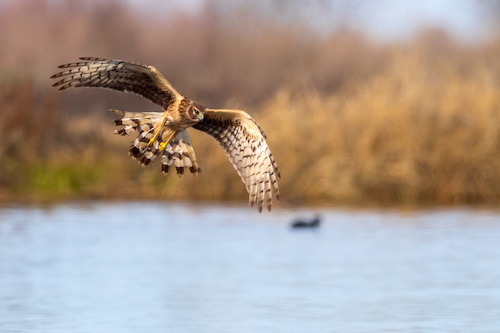This is a professionally captured photograph of a majestic bird of prey, likely an eagle or a hawk, showcasing its impressive wingspan as it flies over a body of water. The bird's beautifully detailed feathers, a mix of brown and light beige colors, stand out against the intentionally blurred backdrop. The composition expertly draws attention to the bird, which appears focused and possibly swooping in on prey. The scene is set in a natural environment, highlighted by light brown reeds and patches of green vegetation along the water's edge. The bright daytime sky visible at the top of the image, combined with the natural lighting, enhances the clarity and vividness of the photograph. No text, copyright, or photographer's name is visible in the image, ensuring the viewer's attention remains on the stunning raptor in flight.